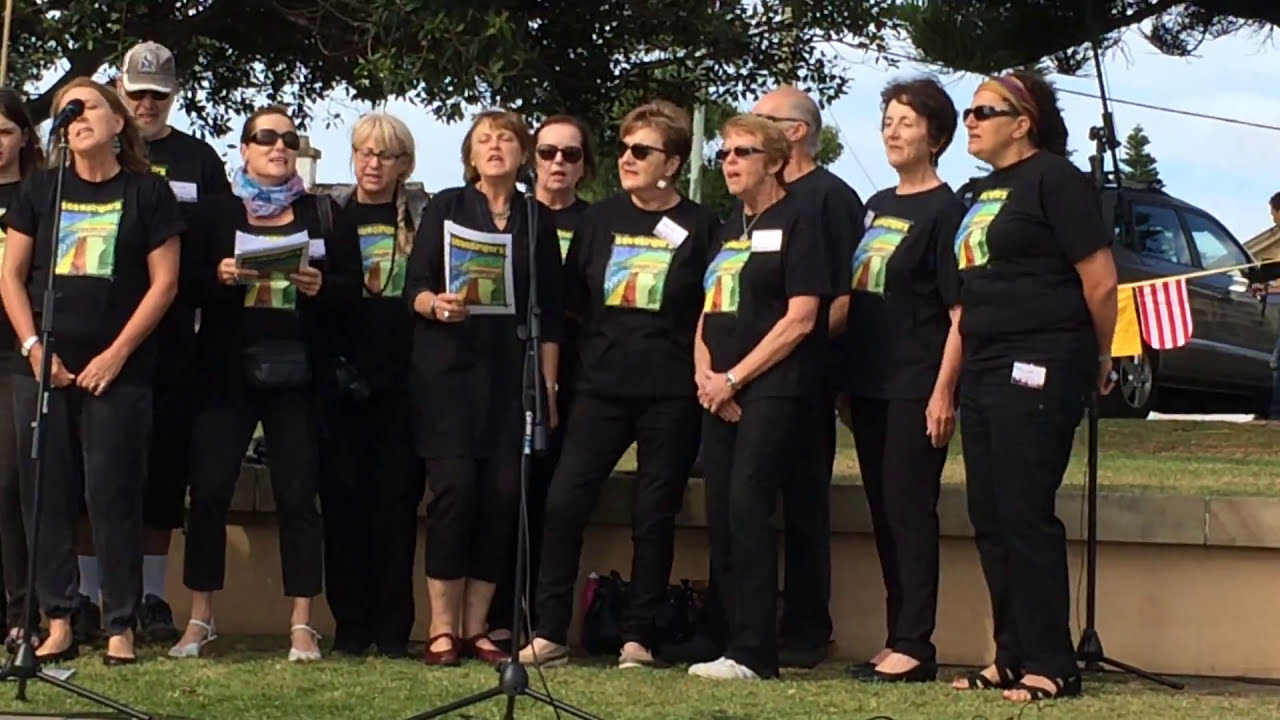In this outdoor image, a group of approximately ten women and two men, all middle-aged adults, are assembled in what appears to be a choir or speaking event. The group, dressed uniformly in black shirts bearing a colorful graphic design of yellow, green, red, and blue hues, stands on a grassy area. The exact details of the design are unclear, but it features elements that could be interpreted as a bridge or tower. Most participants are also wearing black pants, with a mix of full-length and capri styles, and some are sporting sunglasses. 

Three microphones are set up in front of them, indicating that they are singing or speaking. The women at the center and one on the left are actively using the microphones, and some are holding brochures. A car and a small American flag are visible in the background, alongside a tree with green leaves and a string of flags or banners hanging above. They are positioned in front of a short, knee-high stone wall, with more grassy area and trees visible behind them. The man on the left is distinguished by a brown ball cap. The overall setting is serene, enriched by the natural elements surrounding the group.